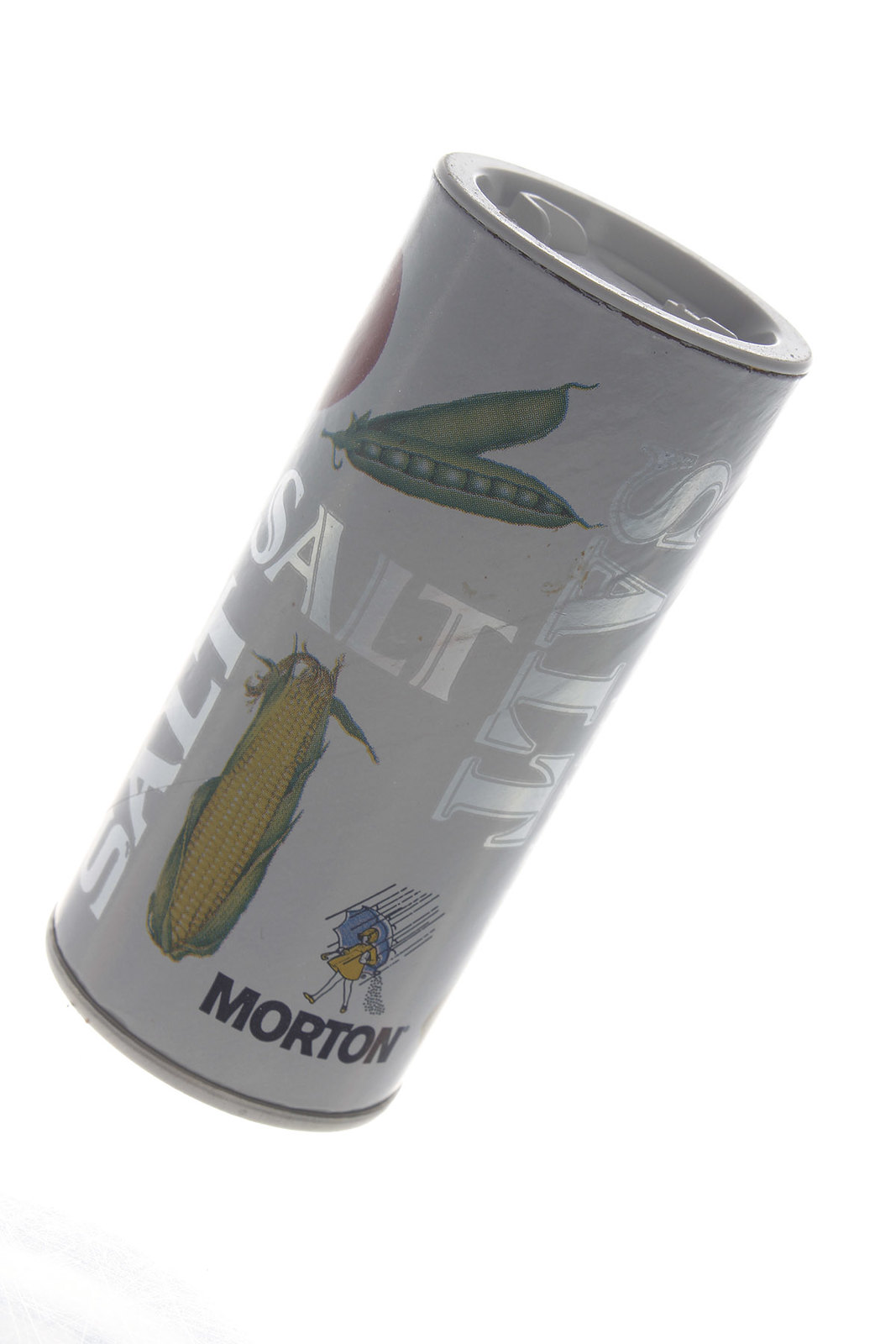The image features a salt shaker prominently displayed against a stark white background devoid of any additional detail. The salt shaker is a self-contained unit, meaning the salt remains within this specific container and is not meant to be transferred elsewhere. It has a cylindrical design, likely constructed from cardboard with a metal bottom for stability. The top of the shaker is made of plastic and can be spun to access the salt inside. The word "salt" is printed in silver and appears multiple times in both horizontal and vertical orientations. The label also includes illustrations of various vegetables. Near the bottom of the shaker, the brand "Morton" is printed, accompanied by the iconic Morton logo depicting a girl in a yellow raincoat holding an umbrella.